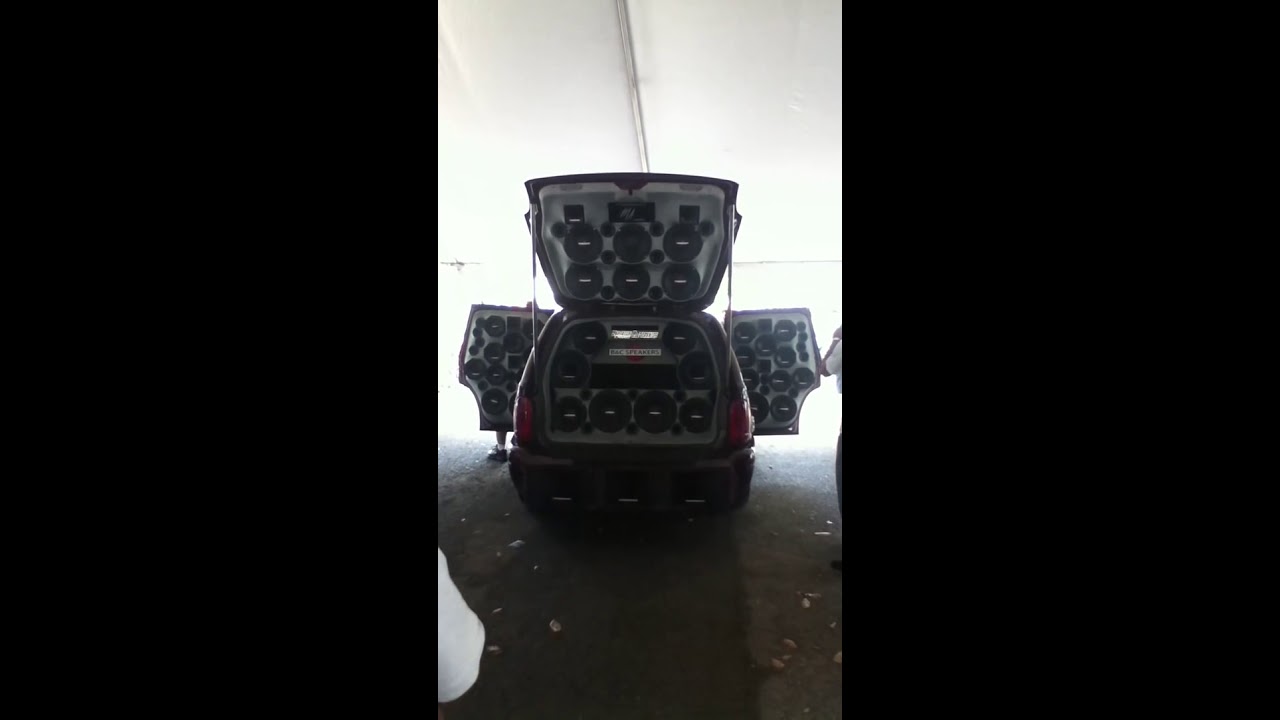The image showcases the rear of a dark-colored van with its back hatch fully open, revealing an interior filled with numerous circular speakers. The back hatch extends skyward, and additional speakers are mounted on the opened doors on both the left and right sides. The van is positioned centrally in the frame, resting on a grayish concrete surface indicative of an indoor structure, possibly a car expo. Distinguishable features include the red, unlit taillights, and black bumpers. A man's arm is visible near the bottom left corner, and another man's legs can be seen under the left-hand door, hinting at human interaction with the vehicle. The environment appears bright and well-lit, possibly by indoor lighting.